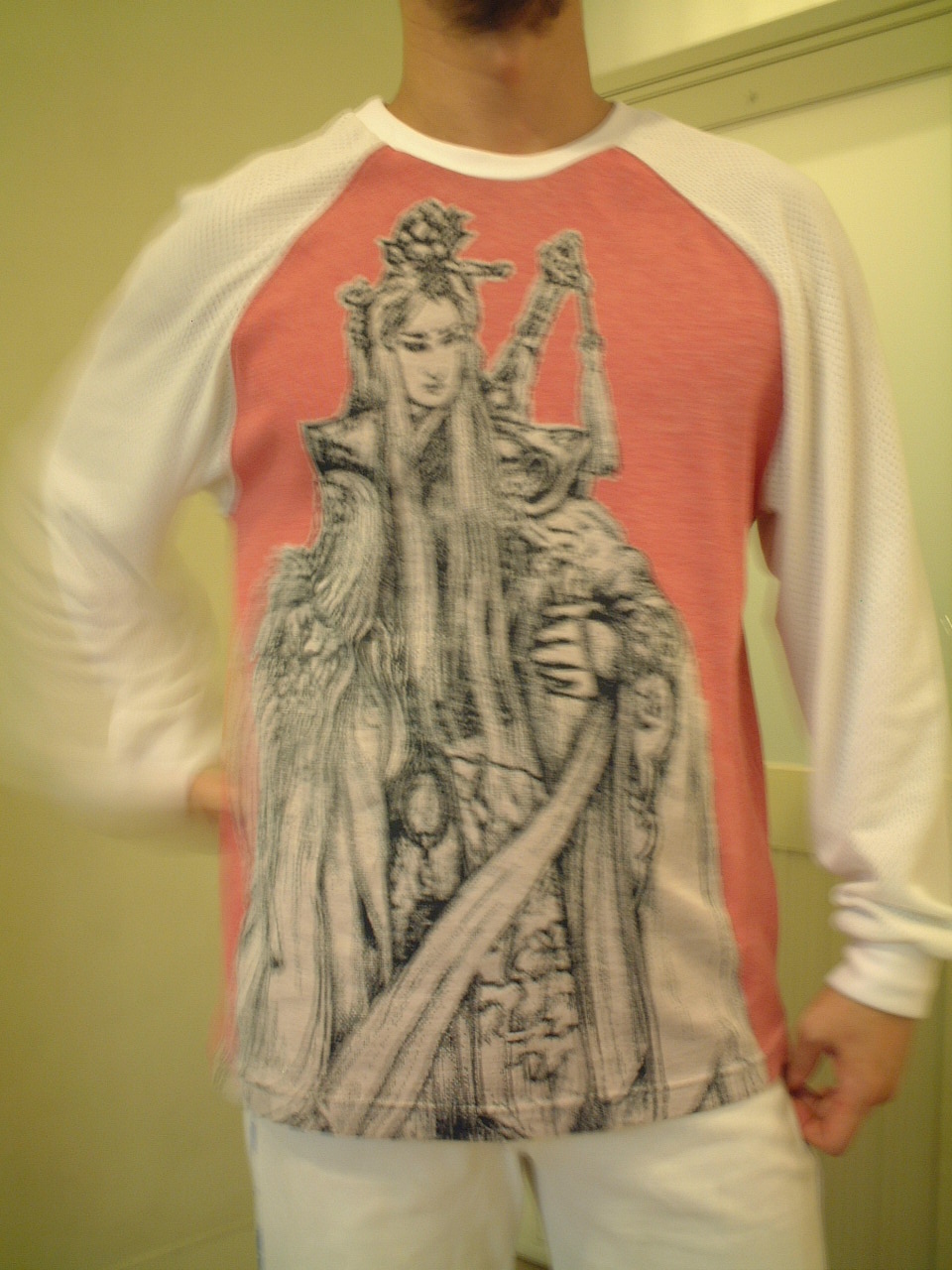The photograph features a man facing directly towards the camera, with the image cut off just below his chin. He has a small beard above his neck, and his Adam's apple is prominent. The man is dressed in a distinctive long-sleeved shirt; the sleeves and collar are white, while the torso is a salmon pink color featuring a black-and-white illustration of a woman in a large puffy dress, with long hair on either side and a pineapple in her hair. The woman holds a crown in her left hand, and a skeleton arm holding a long stick appears in the background of the illustration. The man's right arm is blurred as it moves behind his back, while his left arm rests by his side. He is also wearing white pants. The background consists of a white wall on the left and a white wall with trim at the top and bottom on the right, which is a lighter color.